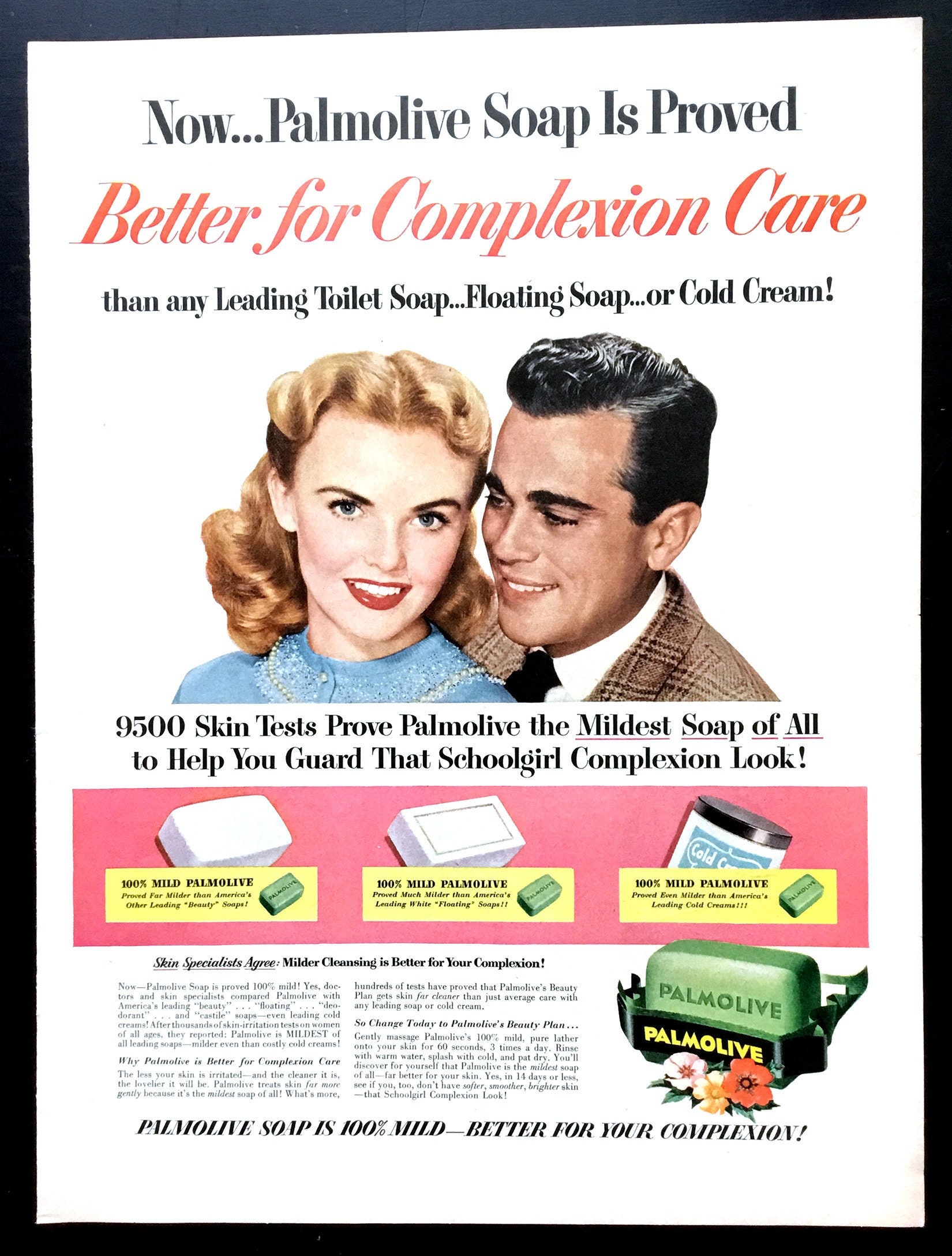This vintage Palmolive Soap advertisement from the late 1950s or early 1960s features a striking layout with a black border surrounding a white background. At the top, bold black text announces, "Now... Palmolive Soap is proved better for complexion care than any leading toilet soap, floating soap, or cold cream!" This declaration is followed closely by eye-catching red italicized text emphasizing, "Better for Complexion Care."

Beneath this headline, the advertisement showcases detailed, colorful drawings of a man and a woman, presented from the shoulders up. The man, positioned on the right, bears a resemblance to Ricky Ricardo with his dark, slicked-back hair, brown skin, and welcoming smile. He is dressed in a brown suit with light brown stripes, a white shirt, and a black tie. On the left, the woman contrasts sharply with her very fair skin, blonde hair parted in the middle, vibrant red lips, and blue eyes.

The next prominent text in black declares, "9,500 skin tests prove Palmolive the mildest soap of all to help you guard that schoolgirl complexion." Below this, a pink rectangular section illustrates three different containers of the soap with unreadable yellow descriptions, symbolizing the variety available. While two additional paragraphs of text are too small to decipher, the bottom of the advertisement reiterates in bold black text, "Palmolive Soap is 100% mild—better for your complexion."

In the bottom right corner, there's a realistic depiction of a green bar of Palmolive soap encased in a black container, labeled "Palmolive" in dark green. Below this, the name "Palmolive" is repeated in yellow, accompanied by illustrations of three flowers in pink, yellow, and red, adding a touch of elegance and freshness to the ad's presentation.